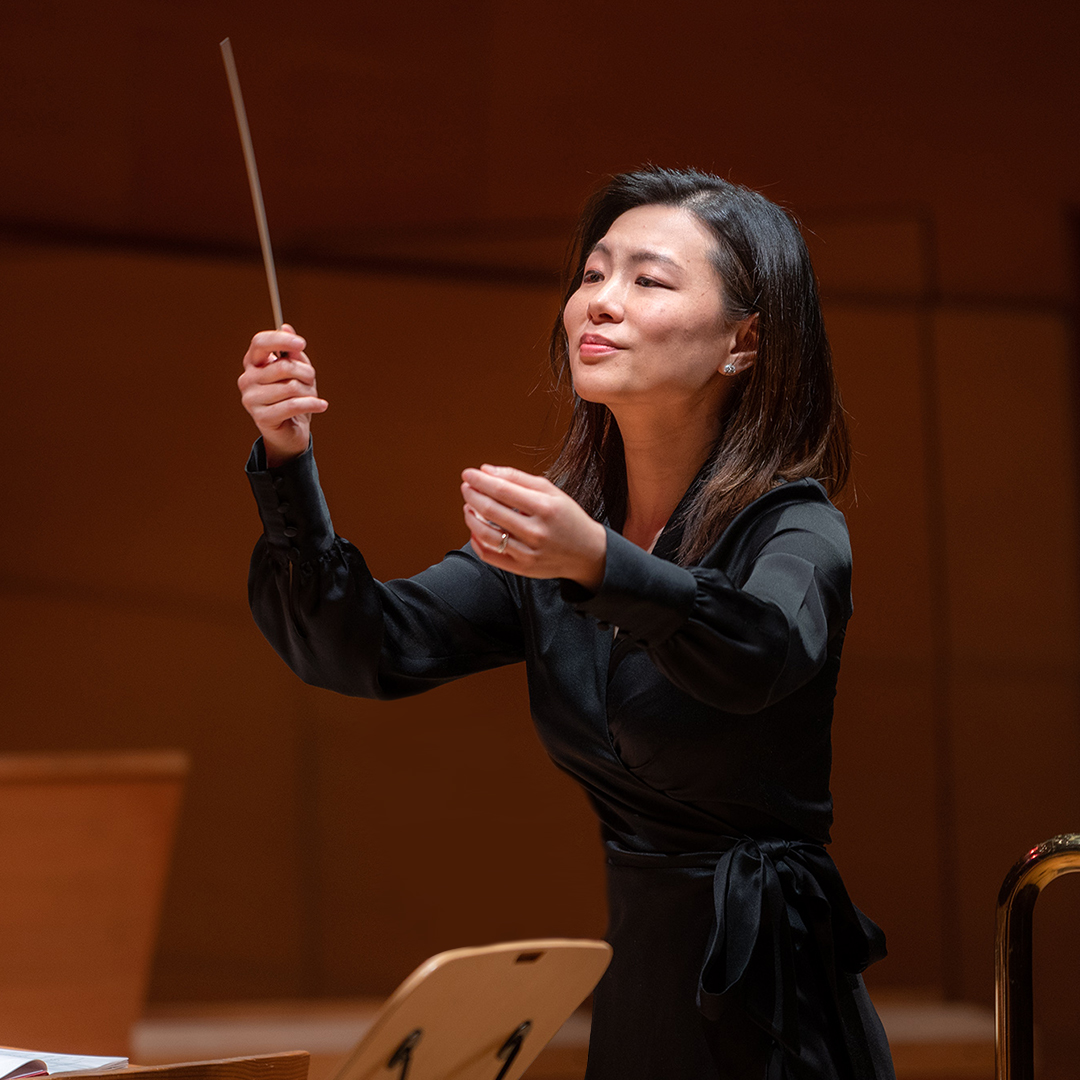This photo captures a distinguished Asian female orchestra conductor in her mid-50s, dramatically lit against the dim, moody backdrop of a concert hall. She stands in profile, facing slightly left, her long brunette hair cascading past her shoulders. Clad in an elegant black dress with a ribbon tied at the waist, she exudes both intensity and grace. Her stern expression and pursed lips highlight her focus as she holds a conductor's baton in her right hand, guiding the orchestra. Her arms are outstretched in a commanding gesture, almost prayer-like in their precision, adorned with a wedding ring on her left hand and sparkling earrings, possibly pearls or diamonds, on her lobes. Below her raised hands, a wooden music stand sits prominently, indicating the score she masterfully directs. The tops of two brown-beige chairs peek into the bottom of the frame, completing the scene of a poised and compelling conductor in mid-performance.